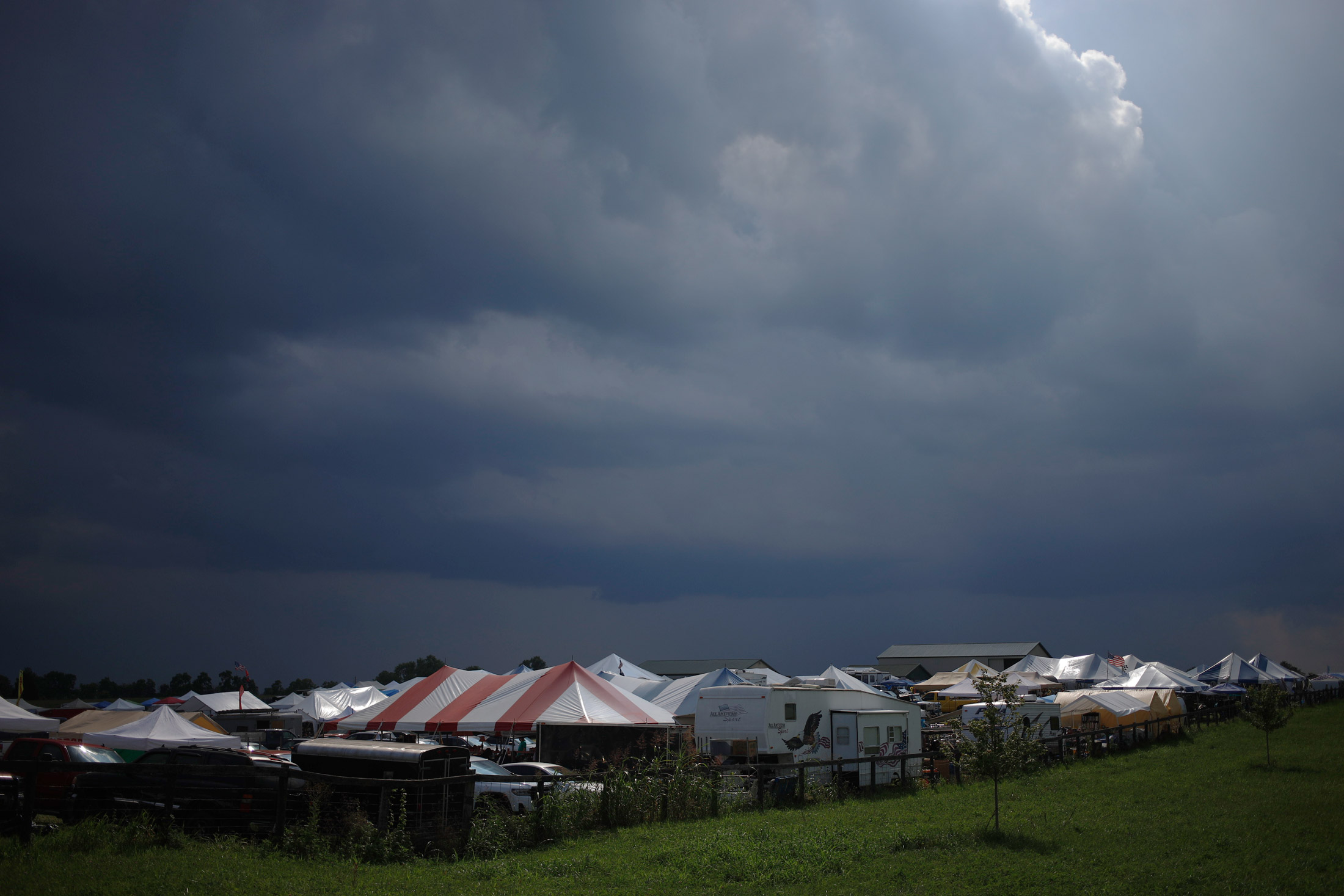The photograph captures a fenced-in fairground filled with a variety of tents, trailers, and cars. The most prominent feature is a red and white striped tent situated in the bottom left corner, adjacent to an RV. Surrounding this main tent are several other tents, including plain white and blue-and-white striped ones. The area is bustling with rows of tents and vehicles set closely together. The fairground is encircled by a grassy field with two recently planted sapling trees situated outside the fenced enclosure. The foreground is framed by more small trees along the perimeter, giving way to the wide-open countryside beyond. The sky above is heavily overcast with dark, stormy clouds that dominate most of the scene, casting an ominous atmosphere. However, in the upper right corner of the image, a small beam of sunlight breaks through the clouds, hinting at a brief respite in the otherwise gloomy weather. The image reveals no presence of people, focusing solely on the occupied fairground against the backdrop of a darkening sky.